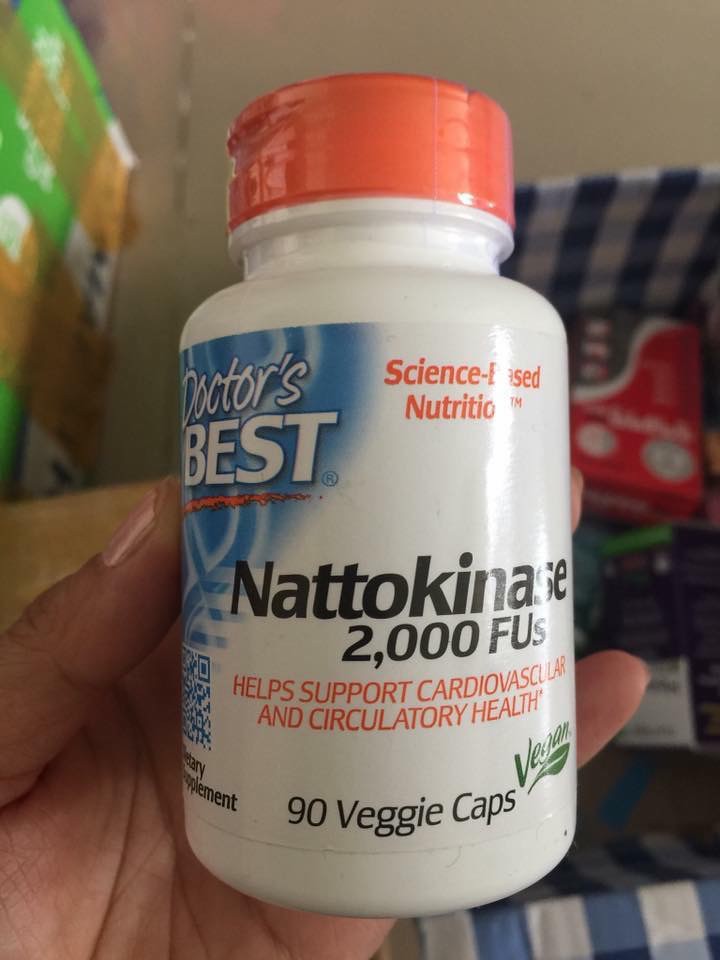A close-up image shows a woman’s hand holding a white, circular plastic bottle of vitamins with an orange cap. The label on the bottle displays the brand name "Doctor's Best" prominently, with "DOCTOR'S" written in white letters on a blue background and "BEST" in bold white letters beneath it. On the right side of the label, in orange letters, the phrase "SCIENCE BASED NUTRITION" is visible. Centered towards the bottom of the label, the product information reads "NATTOKINASE 2000 FUs," followed by the description "HELPS SUPPORT CARDIOVASCULAR AND CIRCULATORY HEALTH" and detailing that the bottle contains "90 VEGGIE CAPS." The background is blurred but hints at some household items, emphasizing the focal point on the vitamin bottle.